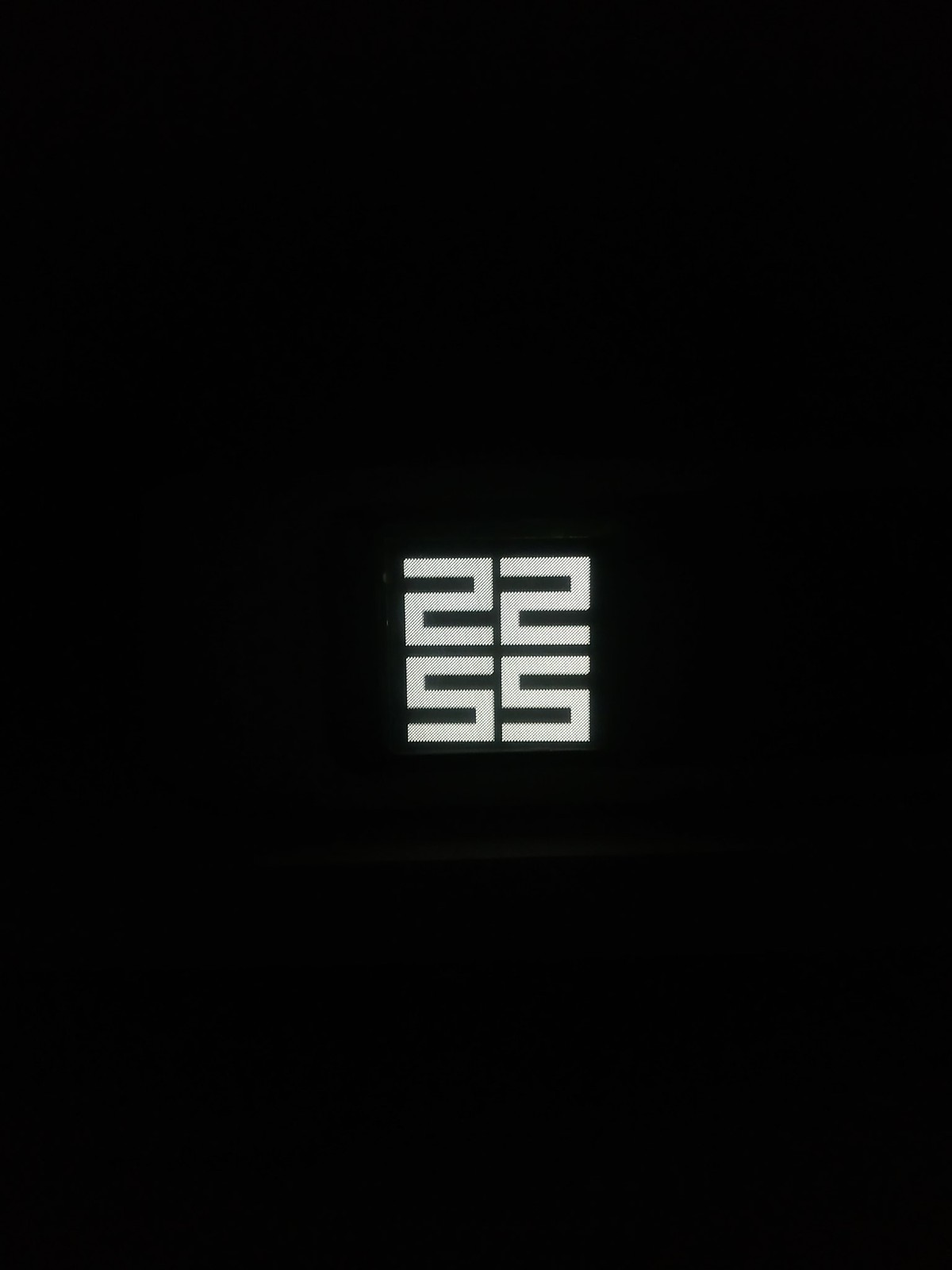The image features a black background with a centrally positioned black cube that subtly protrudes from the backdrop. The cube merges seamlessly with the dark background, but delicate shadows emphasize its edges, creating a slight separation. In the very center of the cube, perfectly aligned white text forms a smaller cube shape with the digits "2 2" stacked above "5 5." The numbers, rendered in precise, straight lines, mirror each other in form and design, showcasing a symmetrical, geometric arrangement.